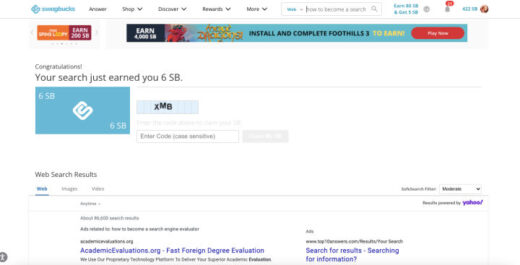Here is a detailed and refined caption for the image described:

"This image showcases the home page of Swagbucks with a clean, white background. In the top left corner, there is the blue Swagbucks emblem followed by 'Swagbucks' written in blue text. Adjacent to this, in black text, are menu options: 'Answer,' 'Shop' with a drop-down tab, 'Discover' with a drop-down tab, 'Rewards' with a drop-down tab, and 'More' with a drop-down tab. Below these, there is a search bar about two inches in length. Above the search bar are two lines of blue text in small font, which are not legible in this image. Next to this, there is a small gray circle and a gray icon with a red circle above it, the details of which are not clear. To the right of this, in red text, there is a monetary amount showing "$32 and some cents" which is partially obscured.

On the left side, there is an orange tab with white text. Below it, a red circle with a red square inside and white lettering that reads 'Earn $200 Swagbucks.' Adjacent to this is a long rectangle with a dark blue left side that reads 'Earn $4,000 Swagbucks,' accompanied by black text that appears to say 'Install and complete foothill three.' Beneath this rectangle, there is a red tab with white text that reads 'Play Now.'

Further down on the left, there is a section that says 'Congratulations' in bold. Underneath, it states 'Your search just earned 6 Swagbucks,' next to a blue square with '6 SB' in the corner and the Swagbucks emblem in the center. Further down, there is another rectangle on the right side that reads 'XMB' in black text. Below this is a long search bar. Underneath, it says 'Web Search Results' on the left, with three clickable options directly below it. On the right, there is another search bar, and below this, there are two paragraphs of black text."